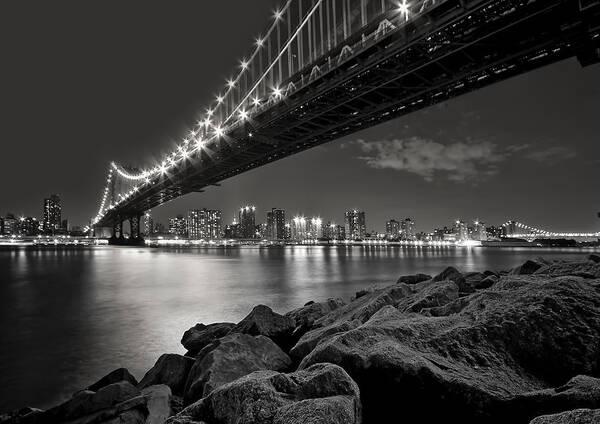This is a detailed black-and-white photograph taken at nighttime, capturing a serene yet vibrant cityscape. The foreground features jagged, massive rocks leading up to a wide, calm river. The water shimmers with reflections from the bright lights strung along a prominent suspension bridge that spans the scene from the top right down to the mid-left. The bridge is dotted with lights, creating a star effect and soft halos, while cables descend vertically from its structure. In the backdrop sits a city skyline with several tall buildings, their windows aglow, adding to the picture's luminance. A secondary, illuminated bridge can be spotted far off to the right. The sky above is mostly clear, marred slightly by a singular puffy cloud, enhancing the moody, tranquil atmosphere of this monochrome image. The perspective from below the bridge allows a striking view of its underbelly, highlighting the interplay between urban architecture and the natural landscape below.